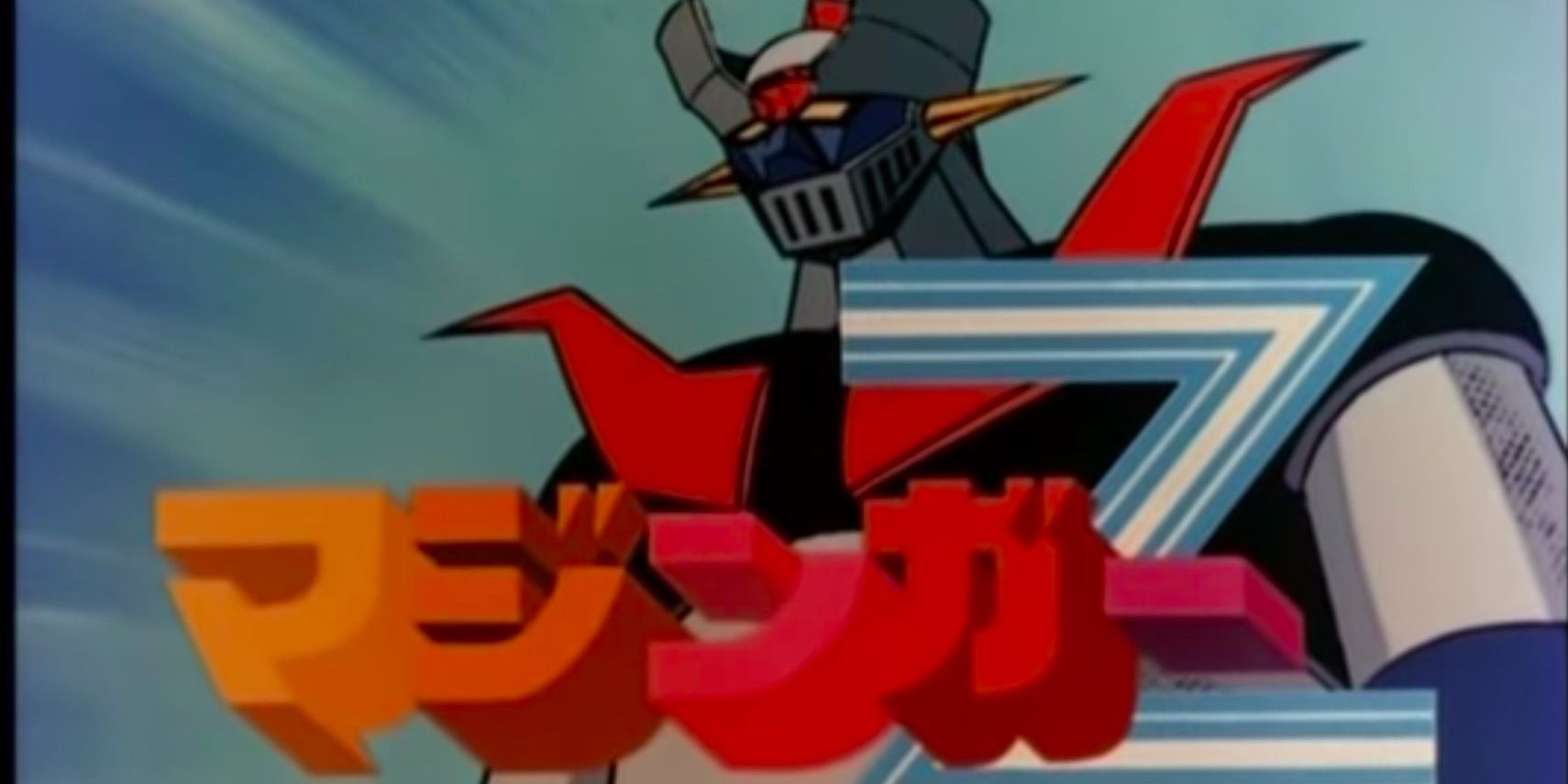This is an opening screen of a Japanese anime cartoon featuring a giant robot reminiscent of characters from series like Transformers or Voltron. The robot stands prominently in the center, characterized by its knight-like helmet with facial armor covering its mouth, sporting yellowish eyes and yellow spikes on the sides, resembling ears. Its helmet is a metallic gray, complemented by a black upper body and white metal arms. The robot also has a striking red breastplate and large red shoulder pads, contrasting with its darker torso. In front of it, there is 3D Japanese kanji in a gradient of colors ranging from deep red, pink, and orange. The background features a sky with dynamic action lines and a radiant light beam transitioning from turquoise blue to a darker blue. This detailed still encapsulates the dramatic flair and intricate design typical of anime robot shows.